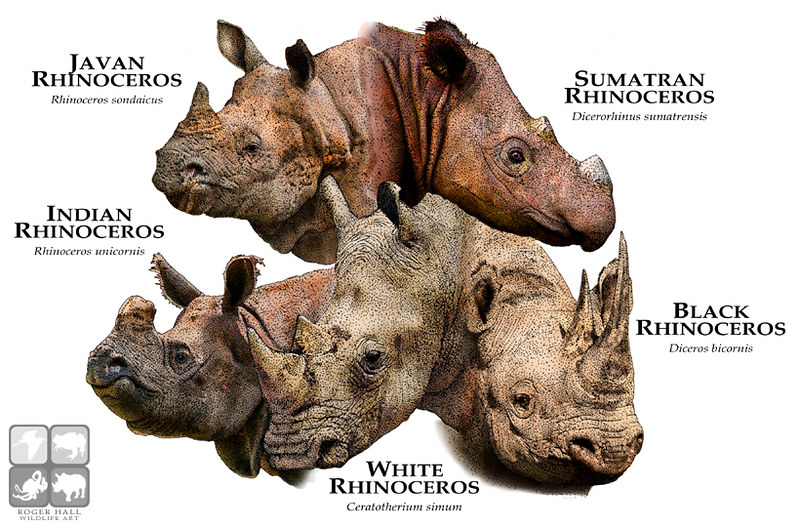The digitally created and photoshopped image serves as an informational collage about rhinoceroses against a completely white background. Central to the composition are the conjoined necks of five different rhinoceros heads, emanating from the middle of the frame and pointing outward. This symmetrical arrangement is accentuated with bold and smaller text labels corresponding to each rhinoceros type. Positioned at various points around the collage, starting from the top left to the bottom right, are the Javan Rhinoceros, the Sumatran Rhinoceros, the Indian Rhinoceros, the White Rhinoceros, and the Black Rhinoceros. Notably, the White Rhinoceros features prominently in the bottom center, including its Latin name, "Ceratotherium simum," below it in smaller text. Each head is oriented in different directions: The two on the top face left and right respectively, while the three on the bottom face left, center-left, and slightly right. Despite their names, all the rhino heads appear in tan to reddish colors rather than their descriptive names. Additional informational labels about the different rhino species, featuring their English names above and their Latin names below, circle around the heads. At the bottom left corner of the image, there is a professional logo that reads "Roger Hall Wildlife Art," emphasizing the educational and artistic nature of the composition.